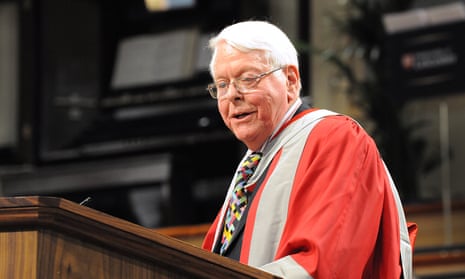In the image, an older man, likely in his mid-70s and somewhat heavyset, stands at a wooden podium, speaking with a gentle smile. He has white hair parted to the left and wears small-framed glasses. Dressed in ceremonial attire indicative of a church or a college graduation, he dons a red robe with gray or white detailing over the shoulders and a multicolored tie featuring black, red, green, blue, and yellow hues. Underneath the robe, he wears a black suit. In the background, a large black pipe organ, partly obscured and out of focus, is visible with an open book on it. On the right side of the image, there is a plant, and behind it, some white text that is too blurry to decipher. A microphone is positioned in front of the man, emphasizing his role as a speaker or leader in this formal setting.